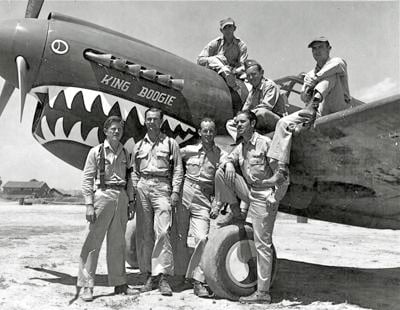This evocative black-and-white World War II-era photograph features seven airmen in beige uniforms posing with a P-40 Warhawk, distinguishable by its prominent shark mouth painting beneath the engine and air scoop. The aircraft, a propeller plane with three blades and visible exhaust ports, is positioned on a beach-like terrain, which appears mostly flat with desert-like qualities. Four of the airmen stand on the ground near the plane, with one placing a foot over the plane's tire. Meanwhile, three others are playfully perched on the aircraft itself—two on the wings and one in front of the canopy. A notable right-side cloud hovers in an otherwise clear sky, contrasting with a large building visible in the left background. This historic photo, likely capturing American pilots, exudes a sense of camaraderie and nostalgia.